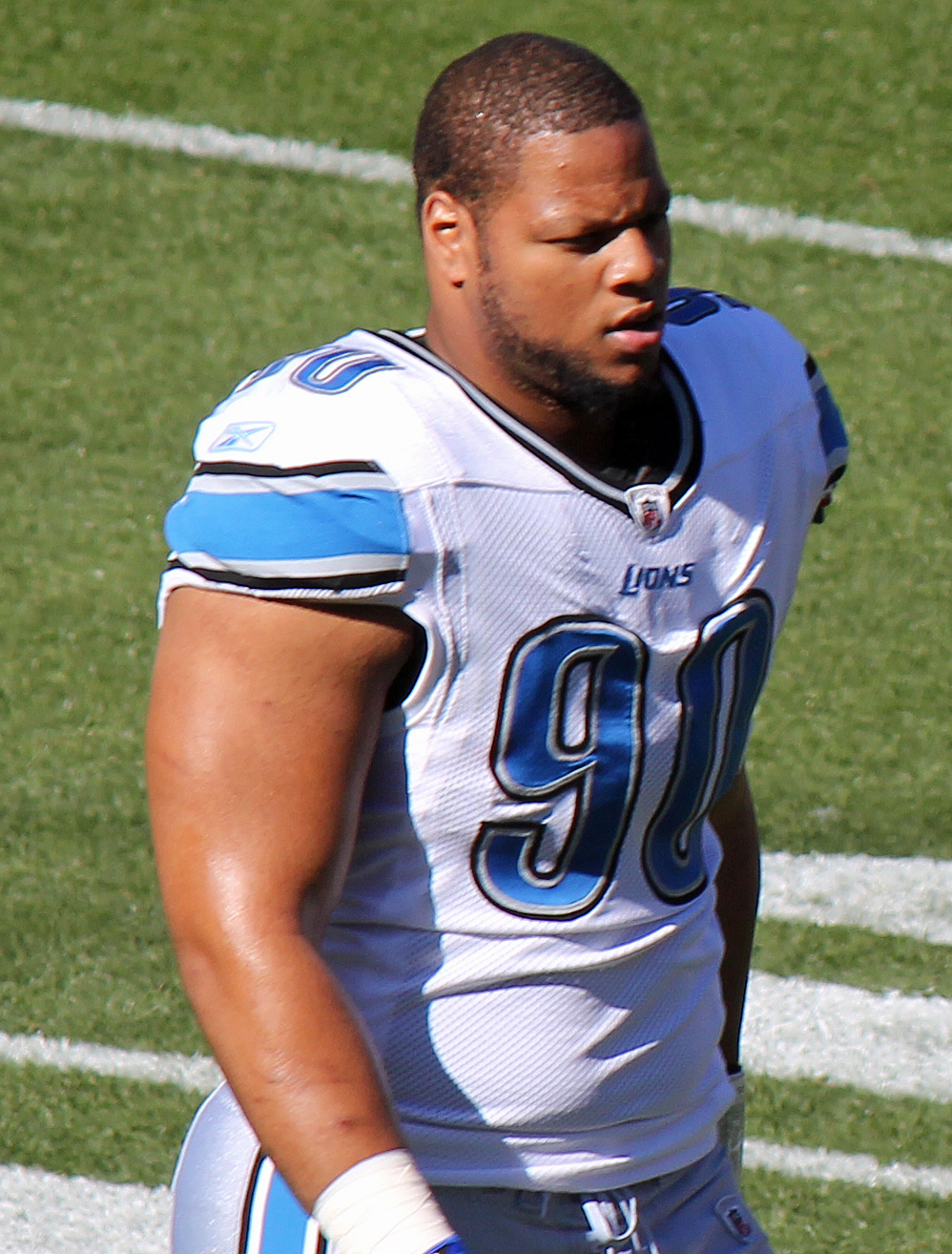In this detailed image, we see football player Ndamukong Suh, who was playing for the Detroit Lions at the time. Suh is captured on a sunny day, standing on a green grass field marked with white lines and numbers indicating the playing area. He sports a white Reebok jersey adorned with the blue number 90 on both the front and shoulders, and the "LIONS" logo prominently displayed on the front in blue letters. The Reebok logo is also visible in blue on his shoulders. Suh is dressed in silver tights featuring a blue stripe and a string on the front, complementing his uniform. His appearance is notable with muscular arms, a white wristband on his wrist, short black hair, and a well-groomed beard juxtaposed by a clean-shaven upper lip, giving him a distinct look. Suh’s arms rest at his sides as he stares towards the left of the image with a semi-serious expression, squinting slightly due to the bright sunlight.